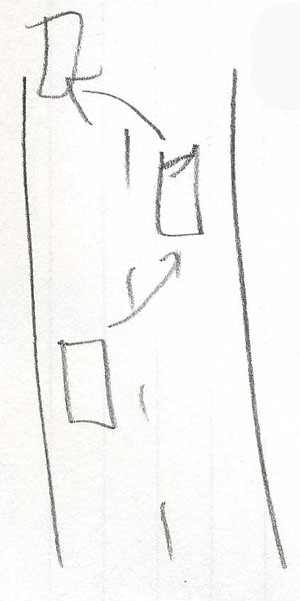The image is a basic pencil sketch illustrating a driving maneuver. Drawn on faintly lined binder paper, the sketch features two solid parallel lines representing the edges of a road, with a series of evenly spaced dots running down the middle, signifying a dotted center line. Situated on this road are three rectangular boxes: two on the left lane and one on the right. Arrows are drawn to indicate the movement of vehicles. One arrow moves from the initial left lane box to the right lane box, suggesting a lane change to pass a vehicle. Another arrow moves from the right lane box back to a further point in the left lane, indicating the completion of the pass by returning to the original lane. The presence of the dotted lines emphasizes that passing is legally permitted on this type of road. The sketch includes no additional colors or details beyond these elements.